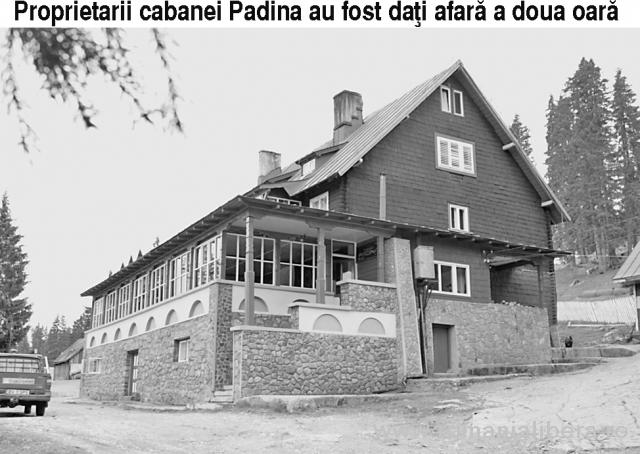This is a horizontally aligned, rectangular, old black and white photograph featuring a multi-story house. The house has a stone foundation with small arches against a white backing on the bottom level and multiple windows, possibly along a porch area. At least two stories are clearly visible, though it is uncertain if the third story's windows are decorative. The building has a hipped roof with two chimneys, and appears to be positioned on a hillside, flanked by tall trees on both sides, against an open sky. An old truck is parked in the far left lower corner of the image, which is indicative of the photo's age. Text above the picture reads: "Proprietary Cabinet Padena, all fast Dati, Afara, Doha, Oara," in black print and without any border surrounding the photograph. The image likely captures a daytime scene in a forested or wooded area, accentuating the rustic style of the house and its surroundings.